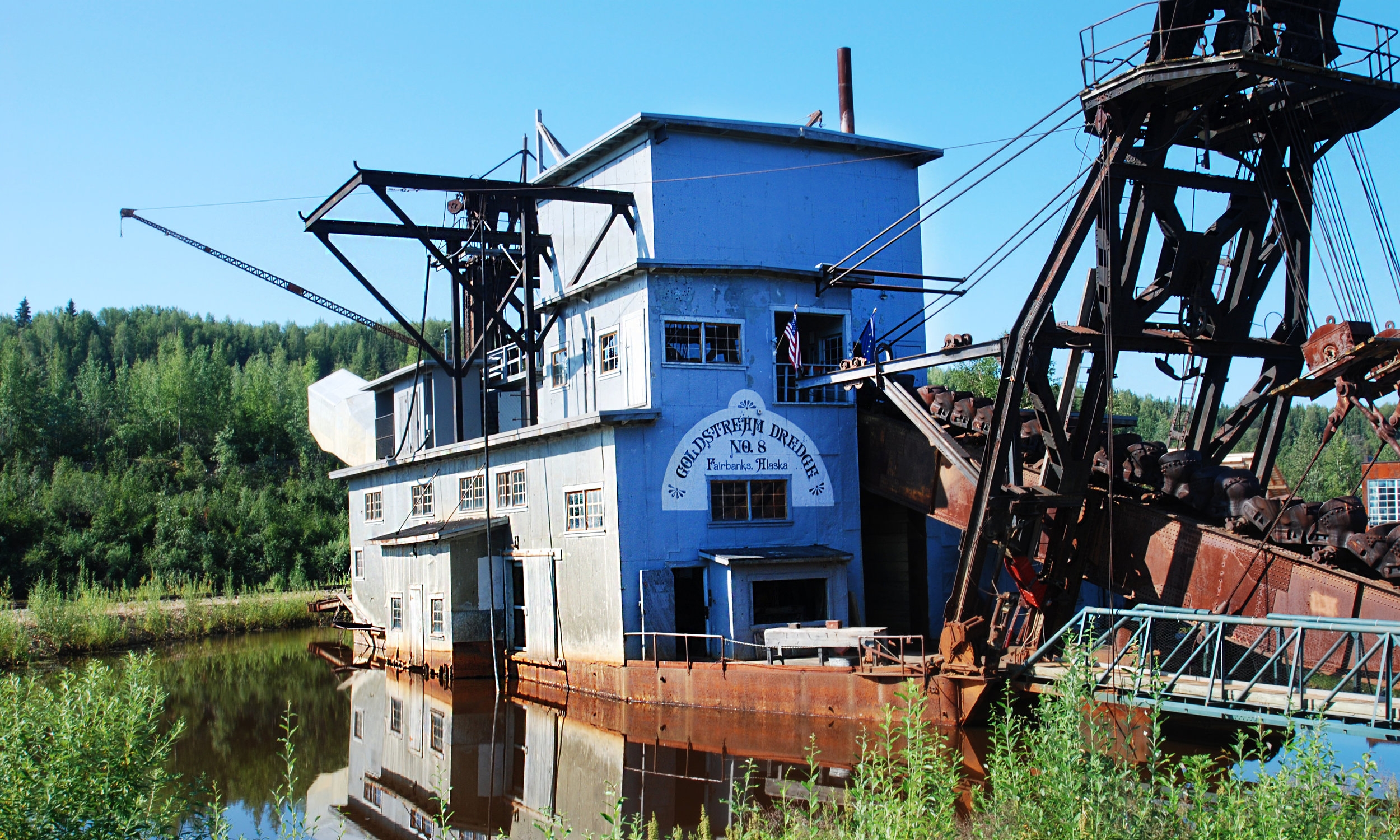This is a well-composed color photograph of a substantial dredging machine named "Goldstream Dredger, Dredge Number 8" located in Fairbanks, Alaska. The image features a large blue building mounted on a rust-colored barge, which appears aged but functional. The building, which has white-framed windows, prominently displays a sign with black text. The barge is designed for heavy-duty work, evident from the extensive metal I-beams, a long arm with cutting teeth for dredging, and an outstretched crane from the front. The scene is set on a river, bordered by lush greenery including trees and bushes, with a clear blue sky overhead. A gravel road is visible to the left, and a walkway extends from the land to the dredger, providing access. The photograph captures the industrial essence of the dredger amid a serene natural backdrop, with defining elements like the American flag, cables, and metal ramps adding to the intricate details of the machinery's working environment.